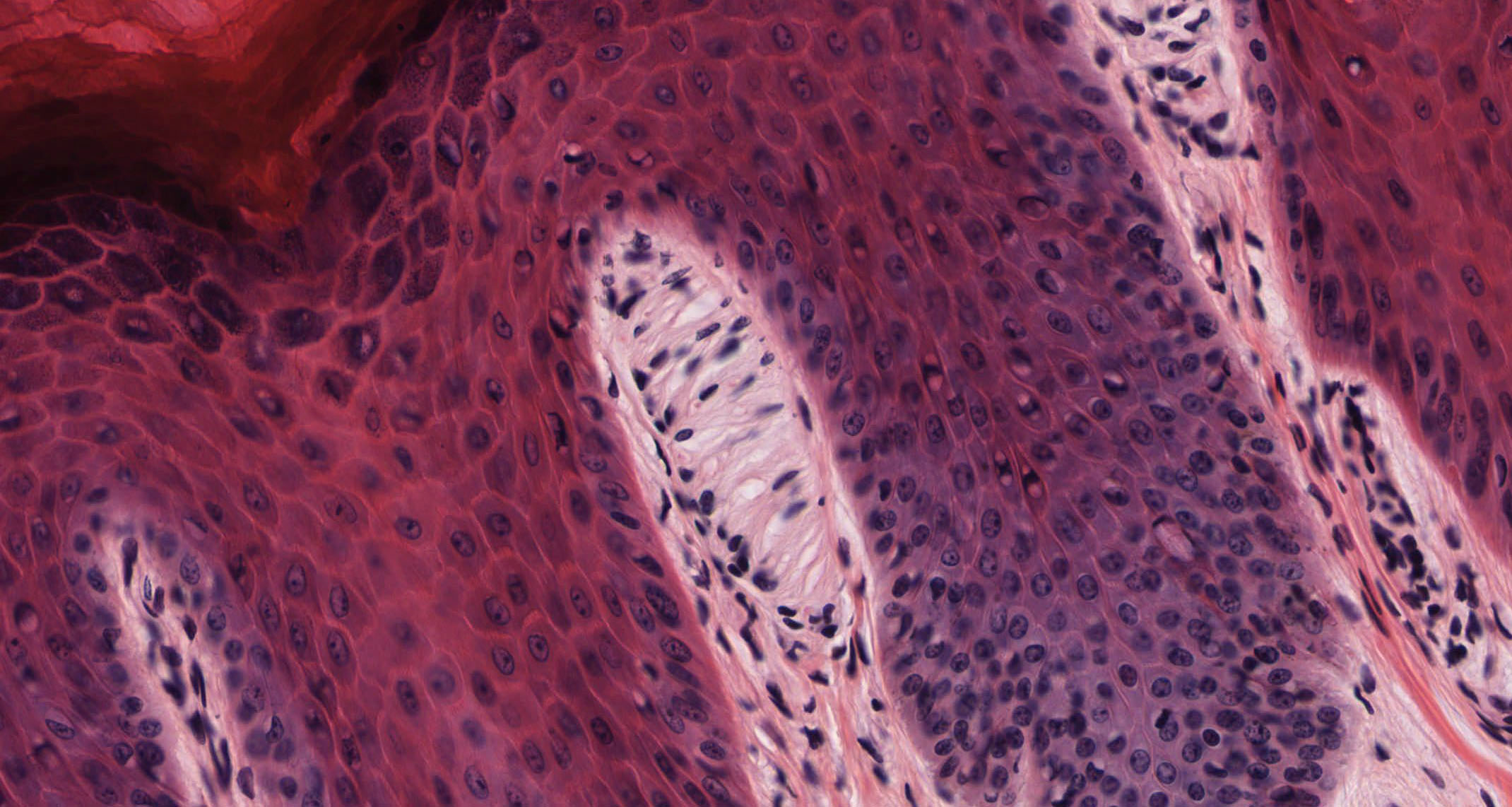This photograph appears to be a highly magnified image possibly taken under a microscope, showcasing the intricate cellular structure of a fruit, reminiscent of a dragon fruit. The image prominently features a series of pink tissues interspersed with numerous small black, seed-like pits throughout. Three distinct white areas traverse the pink tissue, also filled with these pit-like dots, resembling a microscopic viewpoint of the fruit's cellular makeup. On the top left, there is a noticeably different section, more solid and deep red in color, contrasting the surrounding pink and white tissues. This deep red area appears devoid of the seed-like pits present in the rest of the image. The overall scene, with its wavy and abstract patterns, evokes a surreal and detailed glimpse into organic material at a microscopic level.